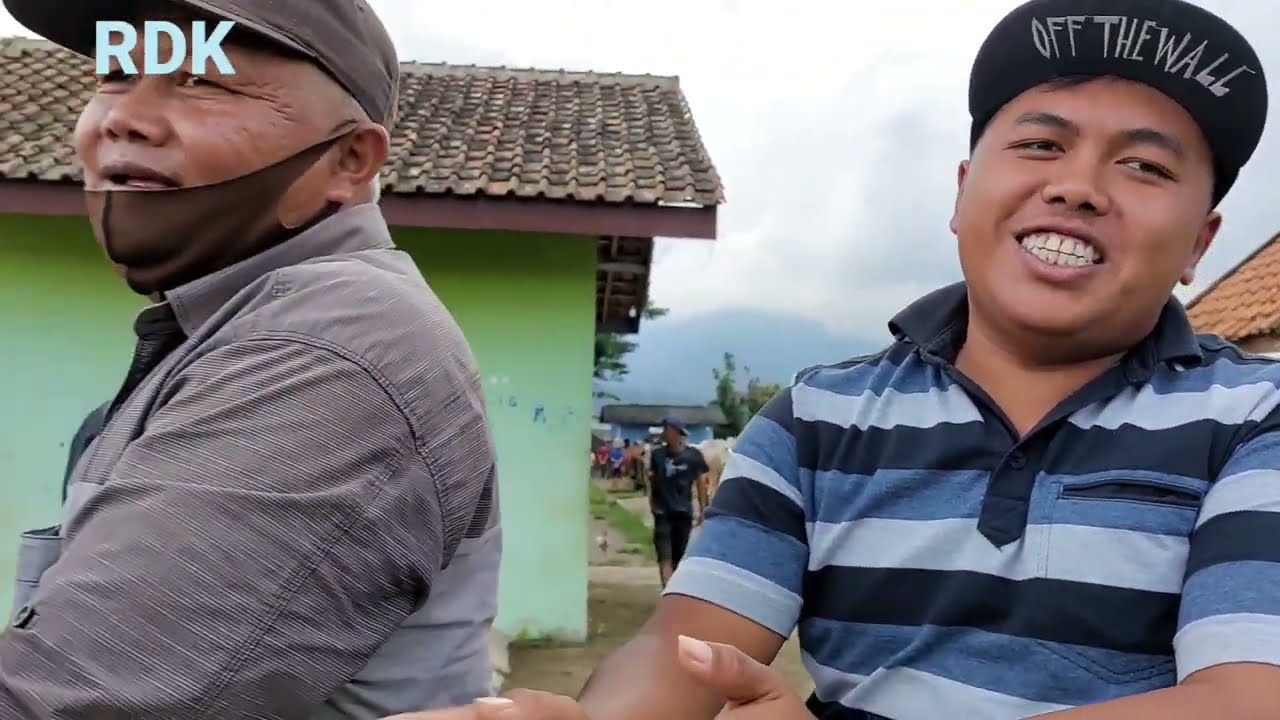This color photograph, in landscape orientation, captures a likely father-son duo front and center. The older man stands on the left, donning a brown cap, a gray button-down shirt, and a brown COVID-19 mask pulled down below his mouth. He's in mid-conversation and looking to the side. Beside him, the younger man, poised with a smile, wears a black baseball cap with the words "OFF THE WALL" in white under the rim, and a striking blue, turquoise, and black striped polo shirt. Their dark skin tones and the intricate details of their attire contrast warmly against the vibrant background.

The scene unfolds in a quaint village, marked by older buildings that suggest a location in Mexico or South America. Immediately behind them, a green house with a brown roof is partially visible, alongside another house with a red roof. Further in the background, a man in a black t-shirt, black hat, and black shorts walks towards them, adding depth to the setting.

In the distance, the architectural vista includes a yellow building with a red tile roof and another structure painted blue with a black roof. The mountain horizon adds a picturesque quality to the photo. The top left corner bears the initials "RDK" in white block letters, hinting at a possible media context like a TV interview.